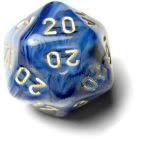The image depicts a slightly blurry and pixelated graphic, likely sourced from PhotoBucket. The focal point is a navy, blue, and gold 20-sided die, featuring a prominently displayed number 20 in gold. The die has a shiny, polished appearance, reminiscent of those used in Dungeons & Dragons games. Near the bottom edge of the die is a thin white strip with navy text, partially obscured and cut off, reading "unlock more of your memories for..." before it becomes illegible. The die casts a shadow on a white surface beneath it, and light reflects off its polished faces. A watermark reading "PhotoBucket" with a cyclone-like icon next to the "P" is overlaid across the center of the die. The image exudes an old, nostalgic charm, amplified by its graininess and pixelation.